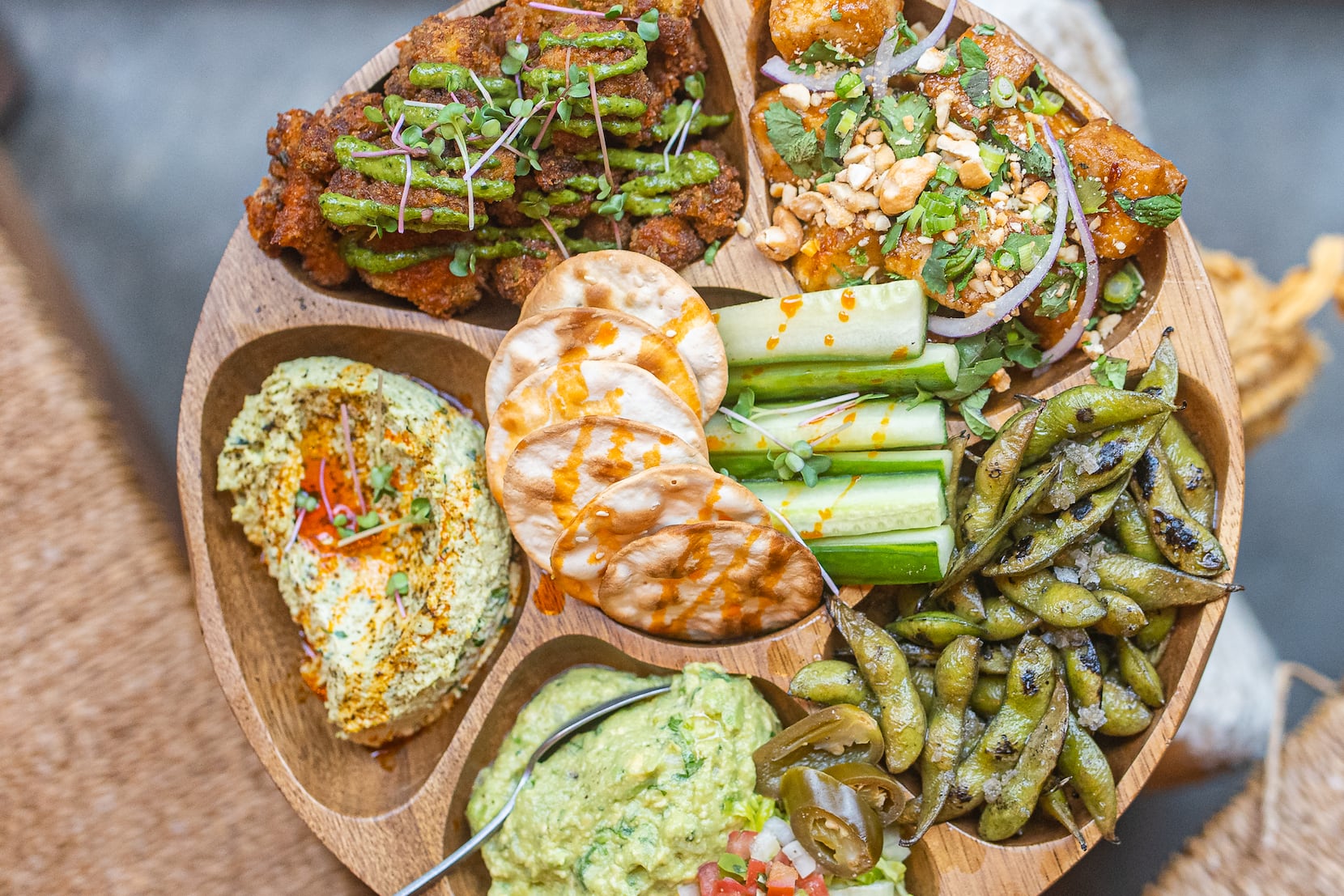This is a close-up color photograph of a unique wooden serving bowl, meticulously divided into six compartments, each containing a variety of foods. The bowl is made of natural wood and features five evenly spaced outer sections with an additional compartment in the center. 

Starting from the top left, around the 11 o'clock position, there appears to be a piece of fried meat or dough, possibly a fried chicken nugget, drizzled with green sauce and garnished with green vegetables. Moving clockwise to the 1 o'clock position, there is browned meat mixed with onions. Continuing around, at the right, there is marbled tofu topped with green onions.

At the bottom, around the 5 o'clock position, we find what might be green lima beans or edamame, possibly seasoned with a sauce. On the lower left, there is a dish that resembles a creamy potato salad with a spoon partially buried in it. At the 9 o'clock position is what appears to be a slice of eggplant garnished with an orange sauce and red powder.

In the central compartment, the bowl contains some round baked chips or crackers accompanied by pieces of chopped celery, all drizzled with an orange sauce. The background is blurred, drawing full attention to the intricately arranged and richly textured selection of foods in this artistic and appetizing presentation.